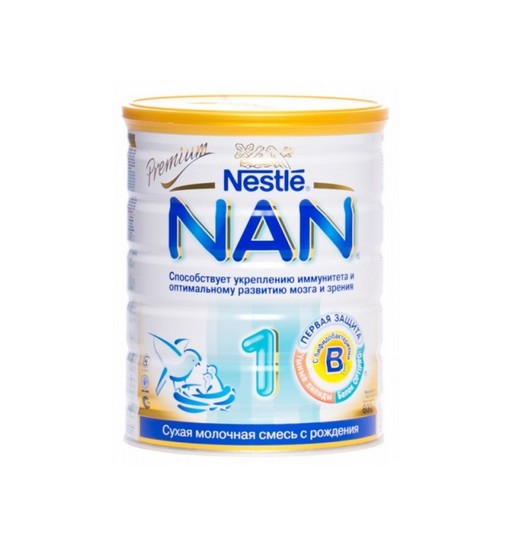The image depicts a cylindrical canister of baby formula labeled in a foreign language. The canister has a yellow lid and a white wrap adorned with various logos and branding elements. Prominently displayed on the wrap in blue lettering is the brand name "Nestle," with "Nan" written just below it. Above the brand name, to the left, the word "premium" is inscribed in cursive and gold lettering. Below "Nan," additional information appears in blue text in the foreign language. Centrally positioned towards the bottom of the canister is a teal oval. Adding to the motherly theme, a small illustration depicts a mother bird feeding her baby birds, suggesting nurturing qualities. Additionally, there is a small yellow stamp on the right side, featuring a blue letter "B" at its center.